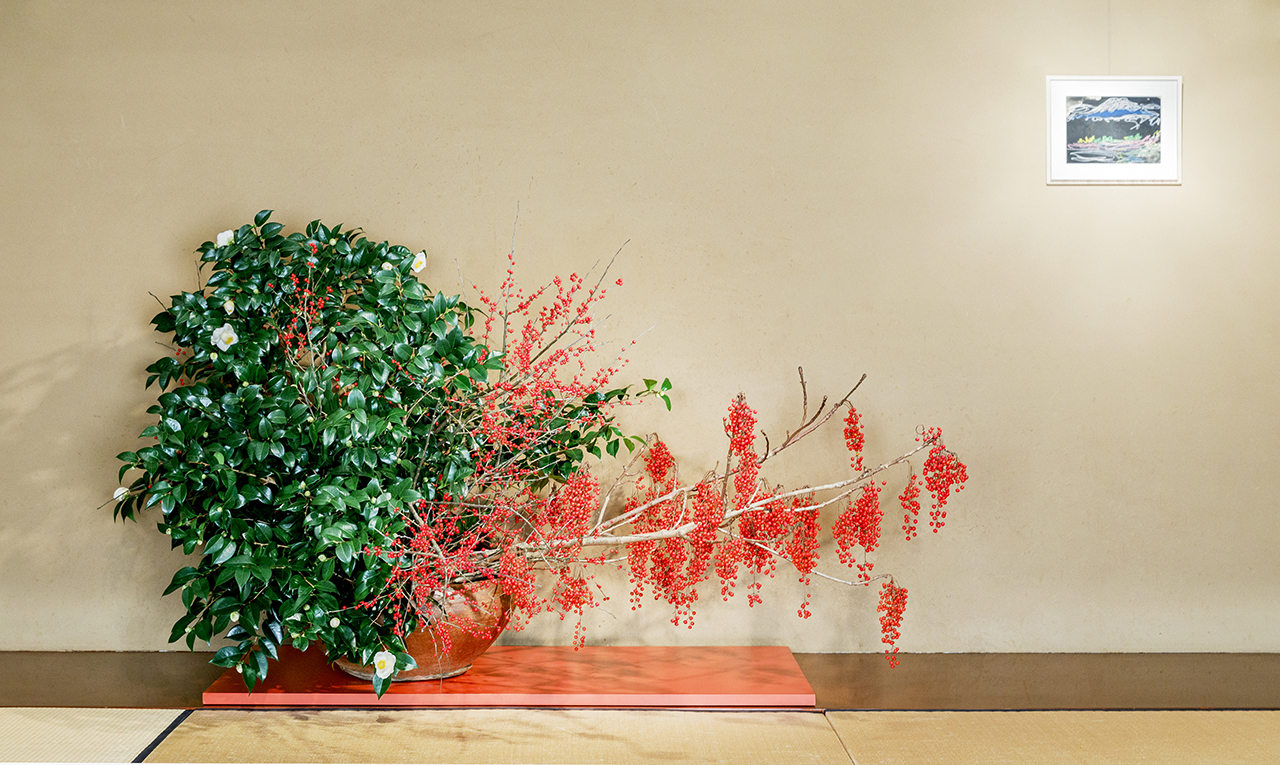The image depicts an indoor scene with a light tan or beige wall in the background. A small white-framed picture showing an outdoor scene with water and mountains is hung on the upper right of the wall. Below, the floor appears to be made of material resembling a mix of dark and light brown tiles, creating a wood-like effect.

In the foreground, a prominent potting container sits on a large red rectangular tile, serving as a base. The container holds a sizable plant with lush green leaves to the left and white flowers. Emerging from the plant, a long branch extends to the right, adorned with numerous small red berries, forming a striking contrast against the greenery. The overall scene combines natural elements with structured indoor decor, providing a visually rich tableau.